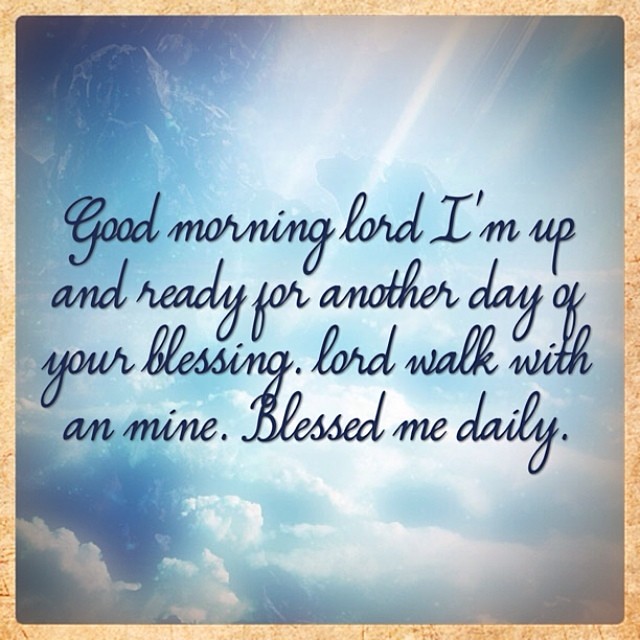This square-shaped Kyoto image features a serene background of blue skies and white clouds pierced by rays of light. Encased in a tan corkboard-style border, the center displays a motivational message written in dark blue cursive over four lines: "Good morning Lord, I am up and ready for another day of your blessing. Lord, walk with me and mine. Bless me daily." The text, though filled with grammatical inconsistencies such as uncapitalized 'lord' and 'your', conveys a heartfelt prayer for daily blessings and guidance. Subtle details, like possible jagged rocks in the top left corner and the overall soothing blue and white theme, add to the image's calming effect.